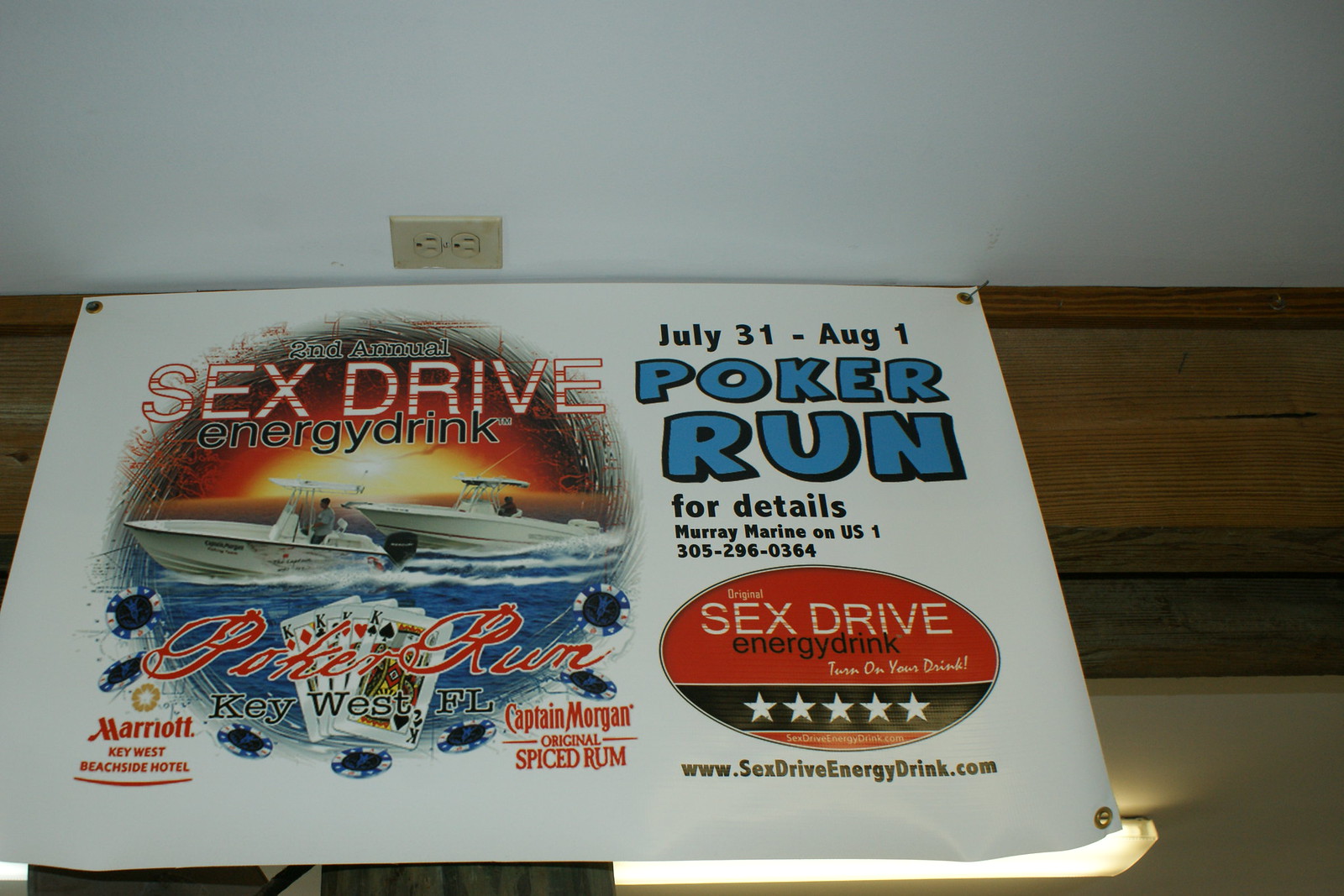The image features a white, slightly reflective banner made from a plastic cloth-like material, prominently hanging from a top rafter. The ceiling it's affixed to is painted white, with a visible power outlet. The banner advertises an energy drink and contains several detailed elements. In the top right corner, dates are listed in black font: "July 31st, August 1st." Below that, in blue font outlined in black, it reads "Poker Run." Further down, in black font, the banner provides contact details: "For details, Murray Marine on US 1, 305-296-0364."

The left side of the banner declares "Second Annual Sex Drive Energy Drink Poker Run, Key West, Florida" and "Marriott Key West Beachside Hotel." There is a detailed circular image of two boats on water with a sunset in the background, accompanied by symbols of poker chips and a deck of cards showing four Kings. Branding for "Captain Morgan Original Spiced Rum" appears prominently. Additionally, an oval with a red background and white lettering reads "Sex Drive," followed by "Energy Drink" in black lettering. Beneath this is the slogan "Turn On Your Diesel" displayed in white letters on a black strip with five white stars, and the URL "www.sexdriveenergydrink.com" at the bottom.